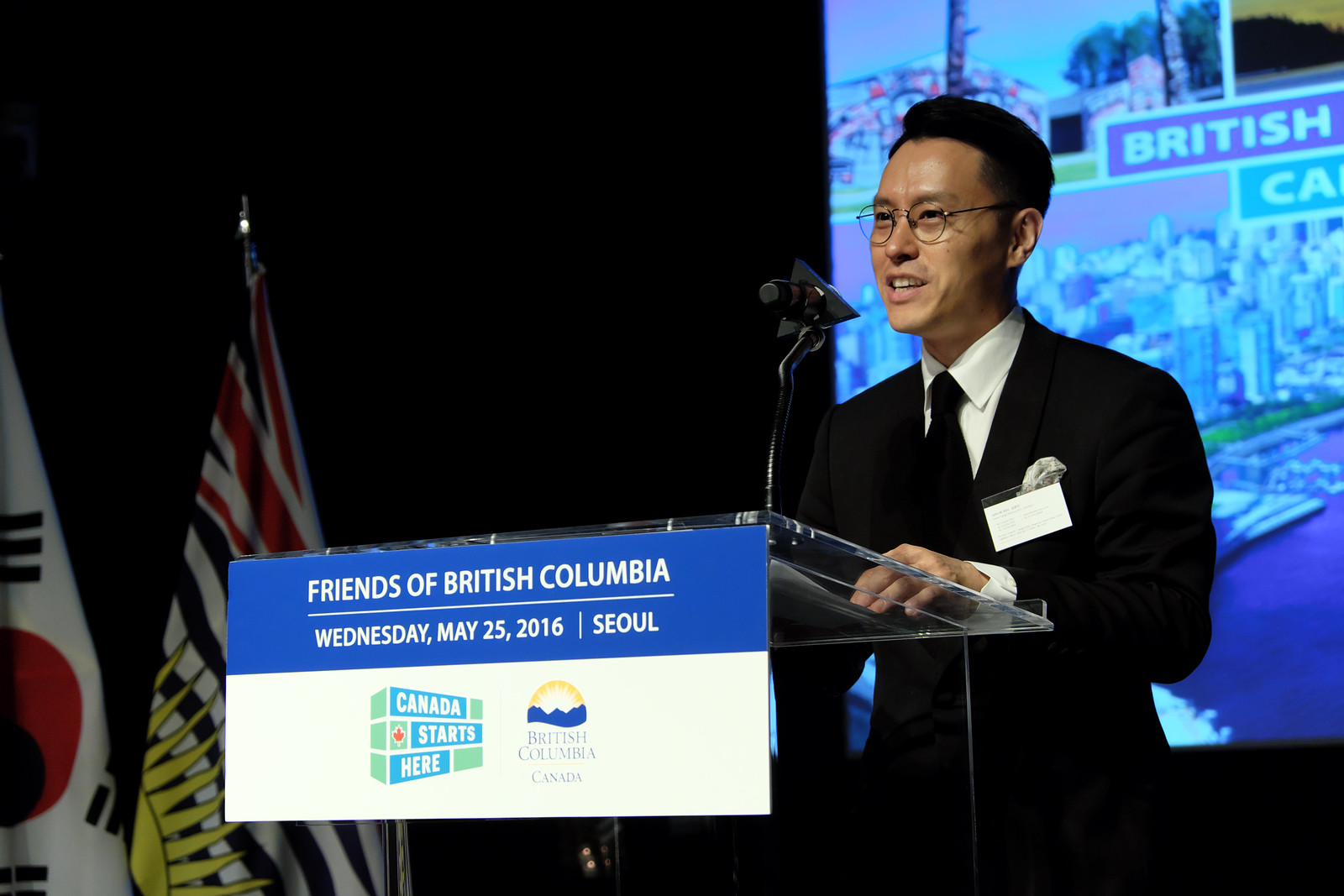The image depicts an Asian man with a lighter skin tone, standing behind a clear podium, his hands resting on it, addressing a crowd. He has neatly trimmed black hair and is wearing wire-rimmed glasses. Dressed in a sharp black suit with a white shirt and black tie, he speaks into a microphone attached to the podium. The podium is transparent, revealing papers placed on top. Attached to the front of the podium is a blue and white sign that reads, "Friends of British Columbia, Wednesday, May 25, 2016, Seoul," and below it, "Canada starts here, British Columbia, Canada." To his left stands two flags, possibly representing different countries. Behind him, a screen displays a partial image of a city along with the cut-off word "British," suggesting it may refer to British Columbia. The entire setting suggests a formal event or meeting.